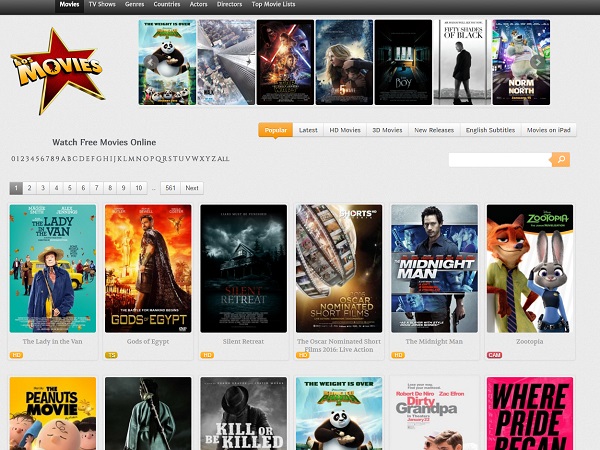The image displays a comprehensive webpage for an online movie streaming site. At the top, a black navigation bar features seven sections: Movies (highlighted), TV Shows, Genres, Countries, Actors, Directors, and Top Movie Lists. An icon reading "Los Movies" is prominently positioned near the top, distinguished by a red star with a gold trim and the word "Movies" in a yellowish-gold font. 

To the right, a selection of movie posters is visible, including identifiable titles such as "Kung Fu Panda," "Star Wars," "Fifty Shades of Black," and "Norm of the North." Below the banner, the text "Watch Free Movies Online" is shown, with alphanumeric navigation options labeled 0-9 and A-Z, alongside an "All" category.

Further down, a row of clickable buttons includes options like Popular (highlighted), Latest HD Movies, 3D Movies, New Releases, English Subtitles, and Movies on iPad. A search bar is also available for users to find specific titles.

On the left side of the page, numerical pagination from 1 through 10 and an ellipsis leading to page 56 is shown, indicating the current view is on the first page. Below this, additional movie titles listed under the Popular section include "The Lady in the Van," "Gods of Egypt," "Silent Retreat," "Oscar Nominated Short Films 2006: Live Action," "The Midnight Man," "Zootopia," "The Peanuts Movie," "Kill or Be Killed," "Kung Fu Panda 2," "Dirty Grandpa," and "Where Pride Began" (partially cut off).

This detailed layout showcases an extensive catalogue of movies organized for user convenience, offering various ways to browse and select films.